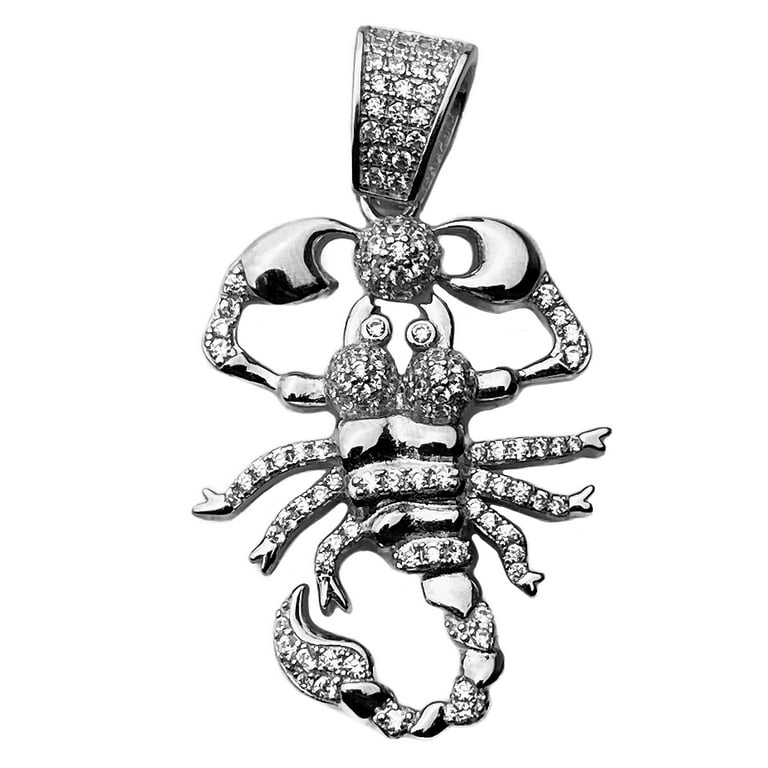This is a detailed, close-up photograph of a sparkling, silver-colored scorpion pendant, likely designed as a piece of jewelry. The scorpion is intricately covered in tiny, shiny rhinestones that resemble diamonds, giving it a luxurious and eye-catching appearance. The pendant features two prominent claws at the front, decorated with rhinestones, as well as a set of six legs adorned similarly. The scorpion's eyes also glimmer with rhinestones, adding to its detailed craftsmanship. The tail of the scorpion is segmented, alternating between the shiny silver metal and rows of rhinestones, culminating in a cluster of rhinestones at the tip. There's a ring at the top of the pendant where it would attach to a chain, although no chain is visible in the image. The zoomed-in nature of the photograph allows for a clear and vivid view of this elaborate and stylized scorpion pendant, emphasizing its artistic and decorative qualities.